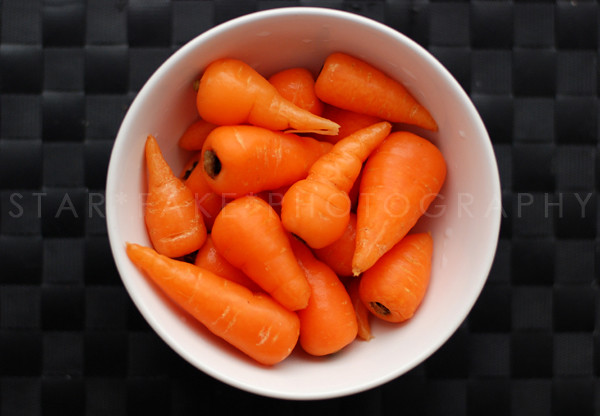In the photograph, a white ceramic bowl, filled to about an inch and a half from the top, contains an assortment of small, fully grown baby carrots. These mini carrots, vividly orange in color, vary slightly in shape and size, with some being wider at the top and tapering to a point at the bottom. The carrots have dark circular marks at the top where their stems were removed, and faint white lines and indentations decorate their surfaces.

The background of the image features a visually interesting checkered pattern consisting of alternating squares of lighter gray and darker black, resembling a woven or felted texture. Superimposed on this background, there is partially obscured white text starting with "S-T-A-R" and ending with "photography," hinting at a possible watermark or brand name "Star [something] Photography." The meticulous details of the carrots and the distinctive background patterns lend a striking contrast and depth to the visual composition.